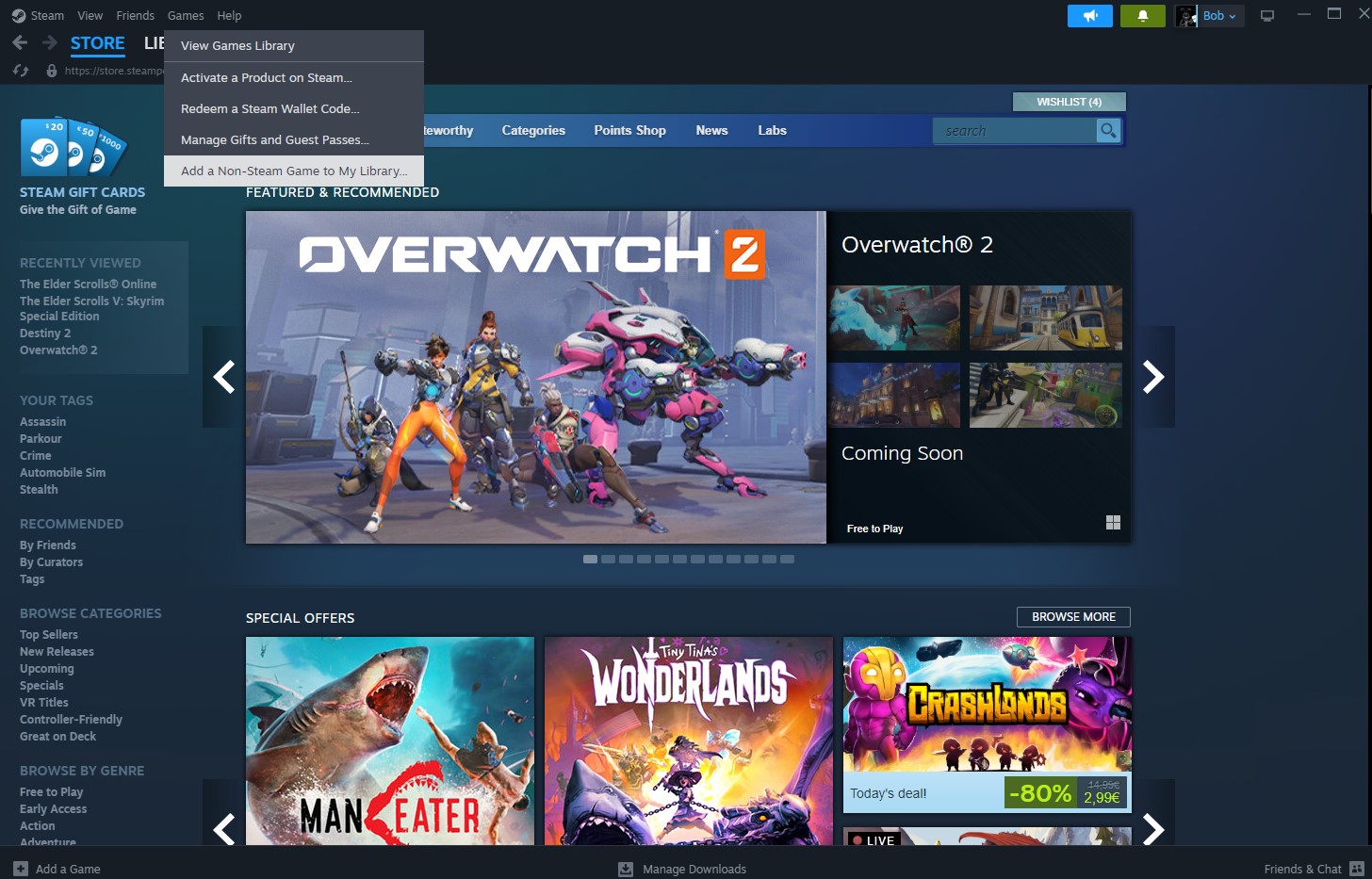This image showcases a screenshot from the Steam store page, the primary digital distribution platform for PC gaming. Dominating the central section of the screenshot is the cover art for "Overwatch 2," featured prominently with additional smaller images of the game. A "Coming Soon" label indicates that this image was taken before the game's release. 

Below the "Overwatch 2" feature is the "Special Offers" section, highlighting several games available at discounted prices. Visible titles include "Maneater," "Tiny Tina's Wonderlands," and "Crashlands," with "Crashlands" specifically marked as being on "Today's Deal" with an 80% discount.

The left side of the screenshot displays a comprehensive menu with multiple browsing options, such as "Browse by Category," "Browse by Genre," "Recommended," "Your Tags," and "Recently Viewed." Additionally, the top left corner features an advertisement for Steam gift cards, showcasing various denominations alongside the slogan "Give the gift of game."